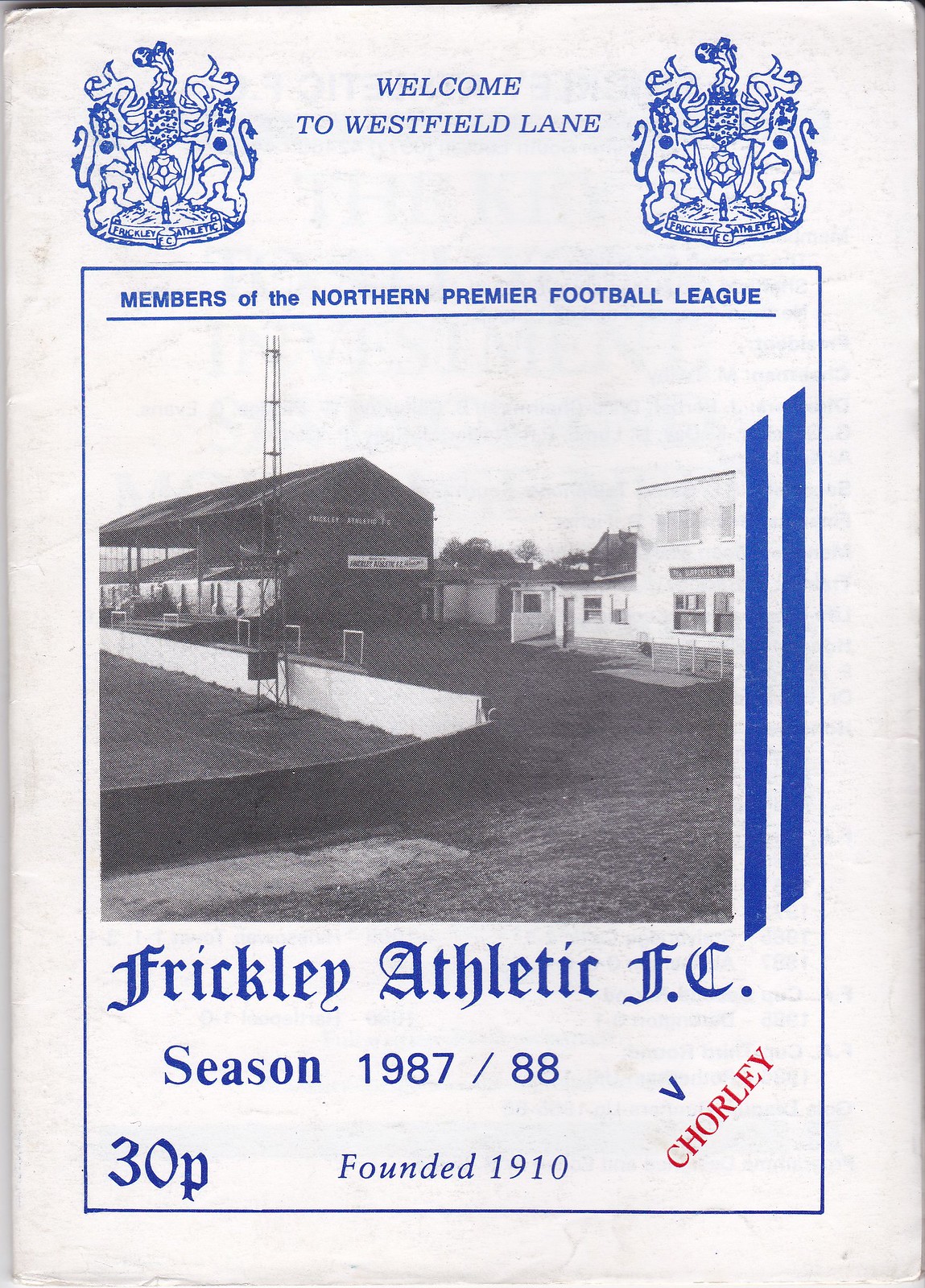The image depicts the cover of a vintage football (soccer) program from the 1987-88 season for Frickley Athletic FC. Set against a white background, the pamphlet features royal blue lettering and accents. At the very top, flanked by two blue crests displaying two lions around a trophy, the text reads, "Welcome to Westfield Lane." Directly below, it states, "Members of the Northern Premier Football League." Enclosed within a dark blue rectangle is a striking black-and-white photograph of a football field, which includes the stands and some surrounding buildings. Under the photograph, bold blue text reads, "Frickley Athletic FC," followed by "Season 1987-88," "30P," and "Founded 1910." Additionally, on the lower right corner, a bold blue 'V' and a red uppercase "CHORLEY" are prominently displayed. The overall appearance of the program suggests it is a relic from the 1980s, highlighting its historic value.